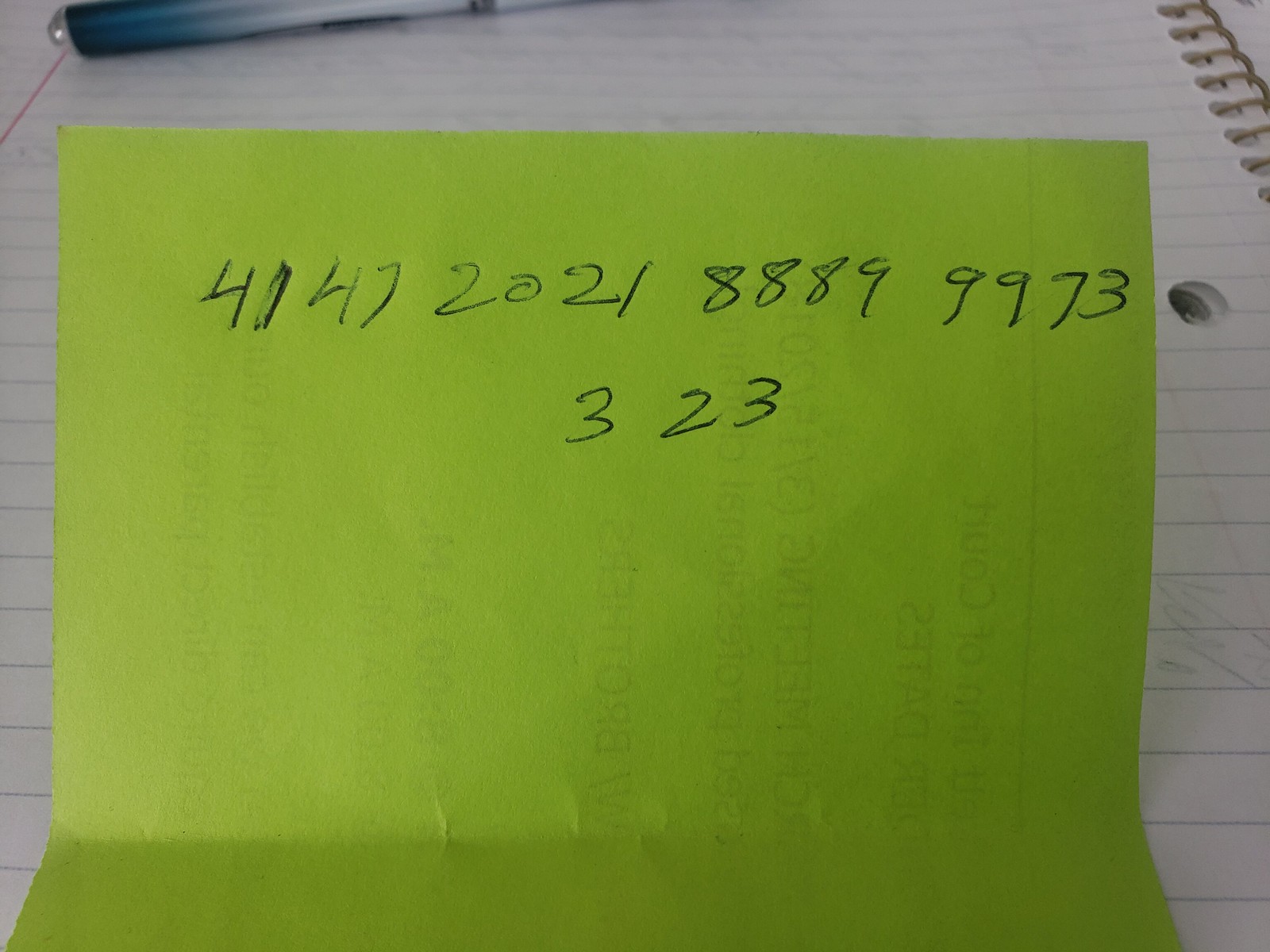A detailed photograph depicts a creased green piece of paper with handwritten numbers, prominently placed atop a spiral-bound notebook featuring lined white paper. In the upper left-hand corner of the image, the top portion of a blue pen is partially visible. The paper showcases a series of numbers written in pen, arranged in two lines. The first line reads "41, 47, 20, 21, 888, 999, 73," while the second line, slightly below the first, displays the numbers "3" followed by a space, and then "23." The paper appears mildly translucent, with some obscure writing faintly visible from its reverse side. The image’s color palette includes shades of green, blue, white, and hints of gray, contributing to a serene and minimalist aesthetic.